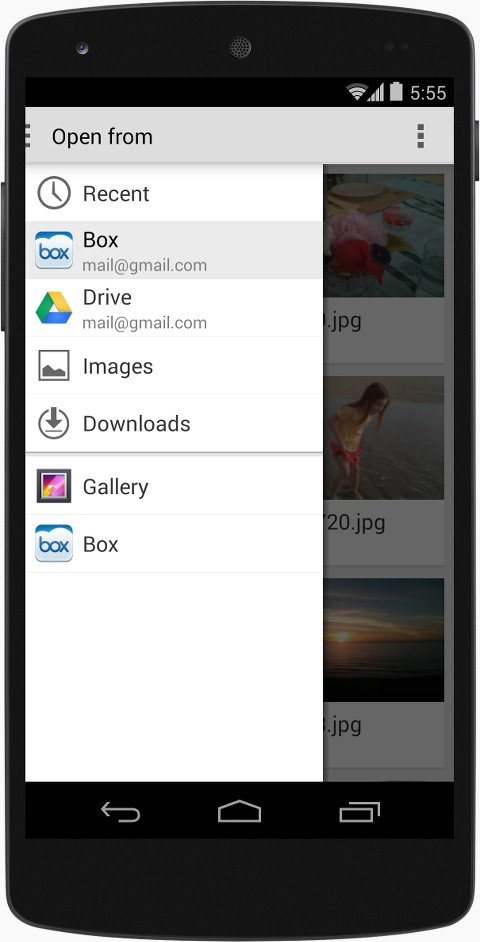A smartphone screen set against a black background displays the time as 5:55. At the top right corner, there are three vertical dots indicating a menu option. The screen shows a thumbnail image of a clock within a blue square, accompanied by icons for "Recent" and "Open" tabs. Surrounding the thumbnail are various app icons: 

- **Mail (Gmail)**: Represented by an envelope with a blue background, and the text "Mail" along with the “gmail.com” domain.
- **Drive**: Depicted by a triangular logo in Google colors (yellow, green, and blue).
- **Images (Gallery)**: A square icon resembling mountains and a circle with a downward arrow, indicating downloads. Next to it, another square shows a purple celestial body, possibly a moon or a planet, set against a cloudy sky.
- **Box**: Featuring an image of clouds and sky with the text "Box."

At the bottom of the phone screen are three navigation buttons:
1. A left-pointing arrow indicating the back function.
2. A circular arrow going to the right and then looping back to the left, signifying the home or main menu.
3. A square shape, likely representing the task view or recent apps.